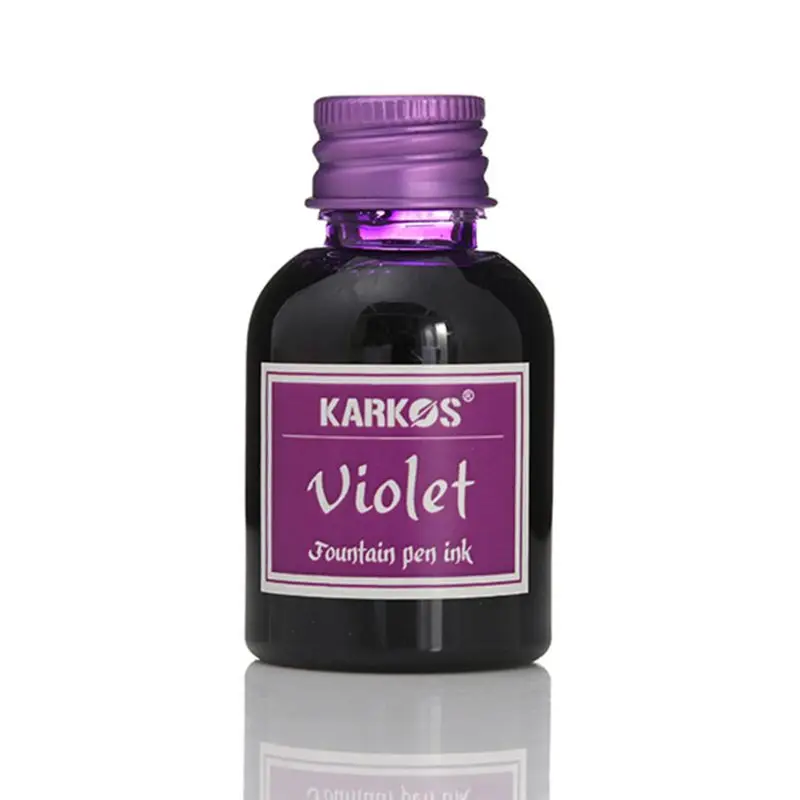The photograph captures a clear, squat glass bottle filled with vibrant violet ink, adorned with a square purple label outlined in white. The label prominently features the Karkos brand name, K-A-R-K-O-S, accompanied by a unique logo of a fountain pen nib crossing the letter O, along with a registered trademark symbol. The words "Violet Fountain Pen Ink" are elegantly written in white script on the label. The bottle is sealed with a screw-on aluminum cap, colored in a matching lavender-purple hue. The reflective surface on which the bottle sits highlights its lower half through its mirrored image, contributing to the bright, pristine aesthetics of the white background. This visually striking setup, likely intended as a product advertisement, emphasizes the rich, inviting color of the ink and the sleek, sophisticated design of the Karkos branding.